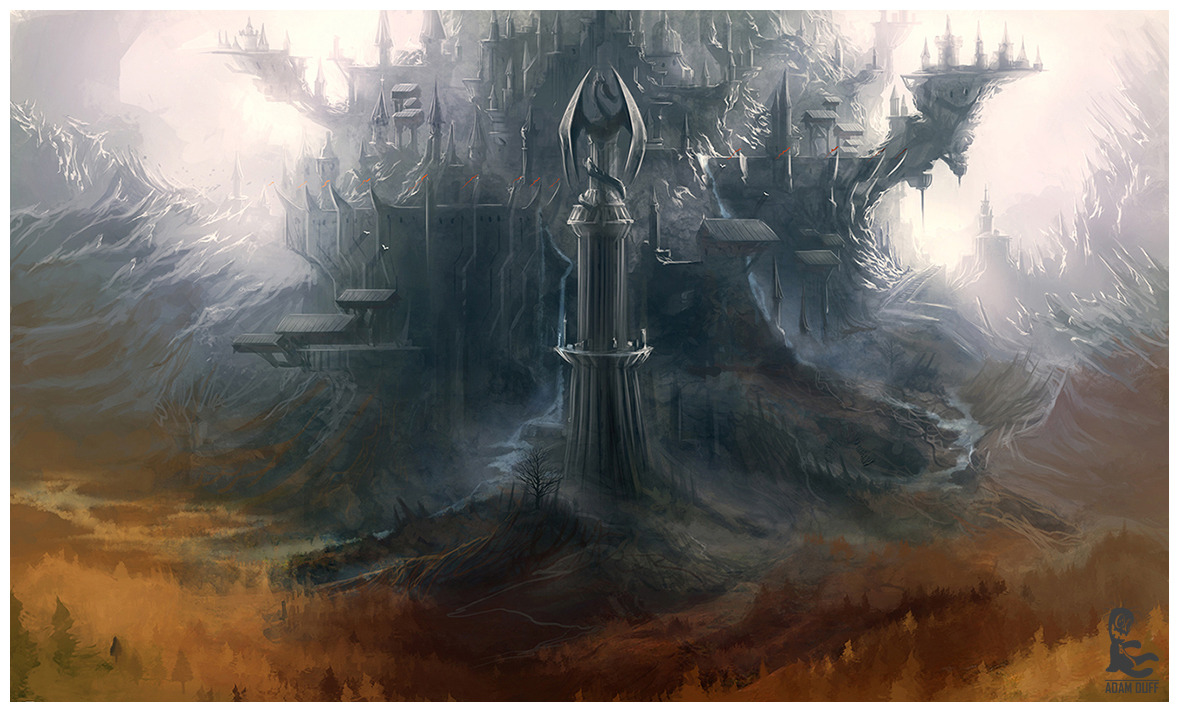This rectangular digital fantasy illustration, wider than it is tall, features a tall, dark, metal tower at its center, crowned with a dragon statue. The dragon, with its wings dramatically outstretched and tail coiled around the structure, faces right and exudes a foreboding presence. The ominous gray and black tower includes a ledge encircling it halfway up and is capped with a steel-like top. In the background, a sprawling, mythical castle with multiple spires and spiky towers adds to the surreal, abstract environment, evoking a sense of dark, brooding mystery, reminiscent of scenes from "Lord of the Rings." The foreground is a blend of oranges, rusts, and browns, suggesting an autumnal, earthen landscape. Light shines luminously from the top of the gray structures, giving the scene an almost otherworldly glow. At the bottom right corner, the artist's signature, "Adam Duff," is visible alongside his logo.